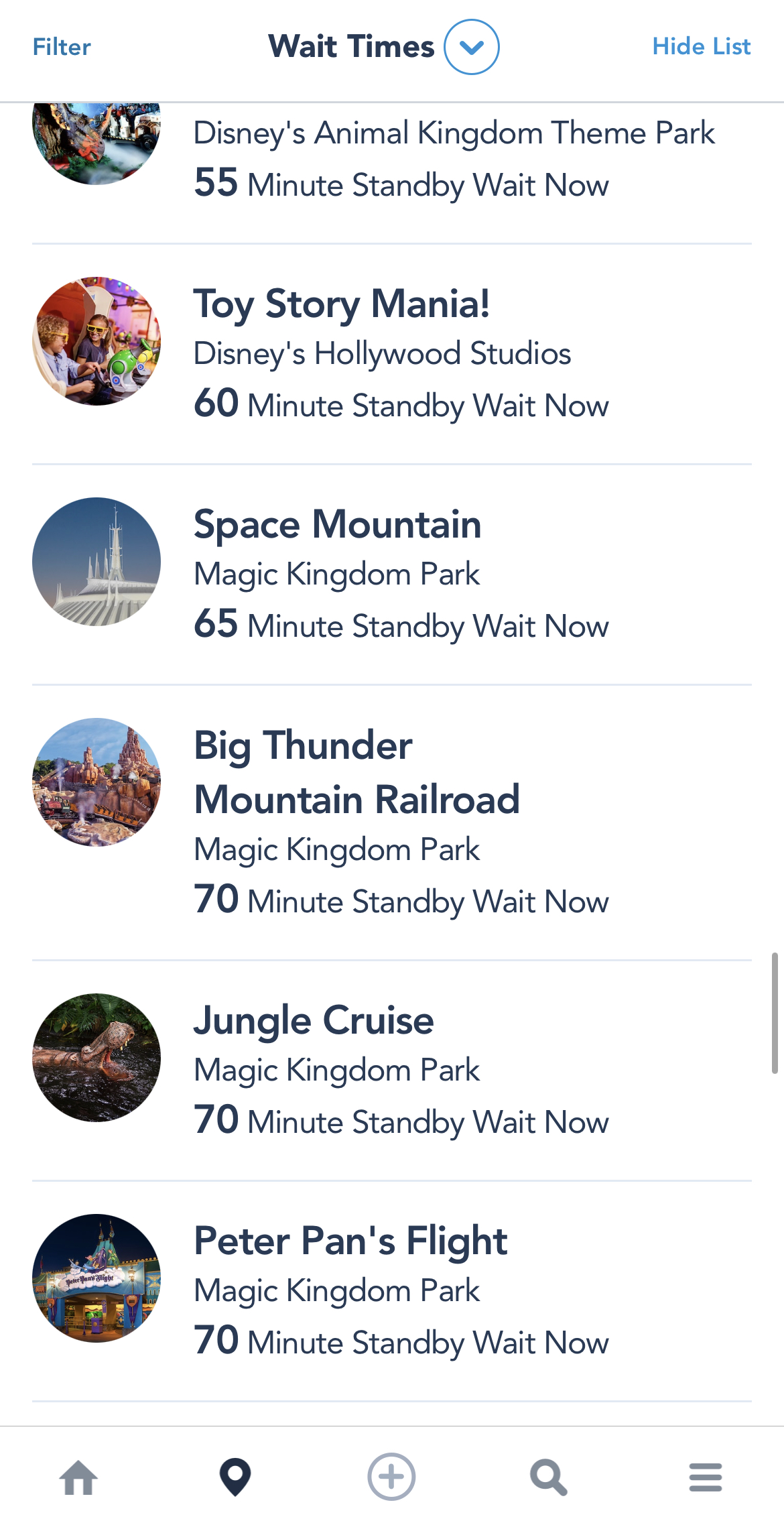The screen capture of the app showcases Disney theme park wait times. At the top, the title "Wait Times" is prominently displayed, flanked by the "Filter" option on the left and "Hide List" option on the right. The list has been scrolled down to reveal various attractions and their current standby wait times. Specifically, Disney's Animal Kingdom theme park shows a 55-minute wait. Toy Story Mania has a 60-minute wait. Space Mountain reveals a 65-minute standby time. Big Thunder Mountain Railroad, Jungle Cruise, and Peter Pan's Flight each have a standby wait of 70 minutes. The overall impression conveys that most rides have substantial waiting periods, suggesting that visitors will spend significant time in lines before experiencing the attractions.